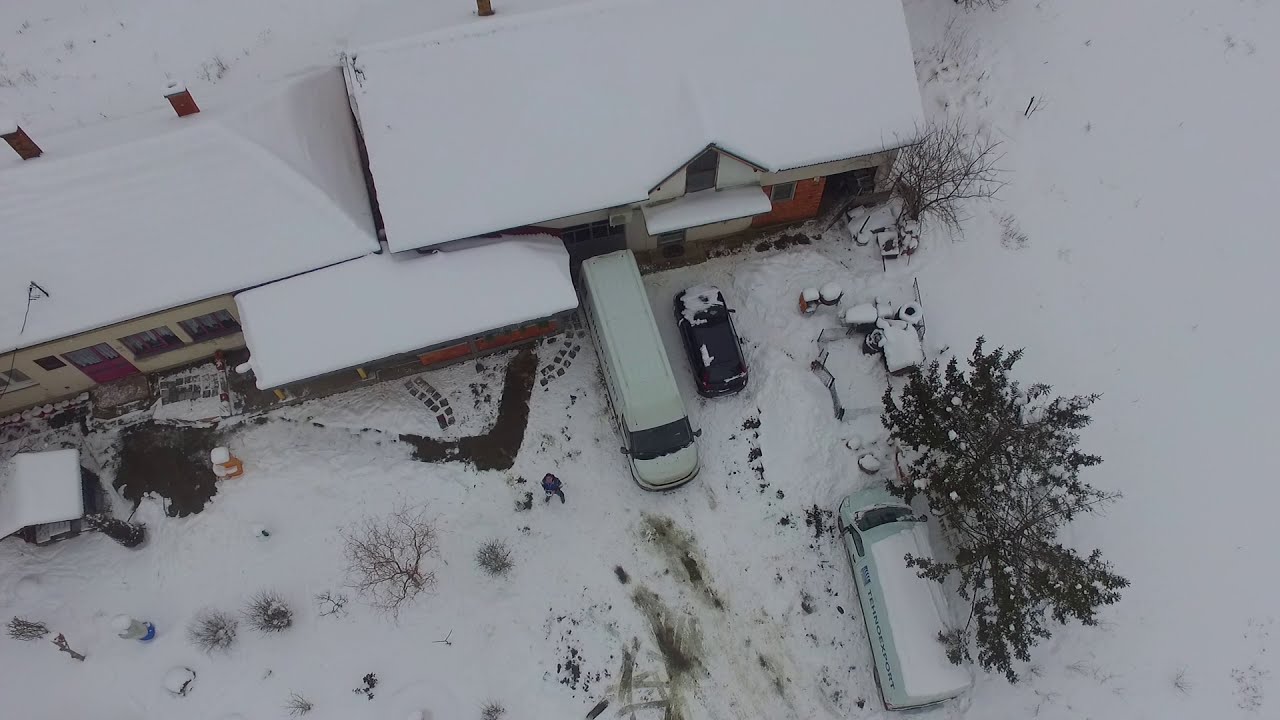This photograph, taken from an aerial bird's eye view, captures a snowy yard of a house during the daytime, bathed in natural light. The ground is blanketed in white snow, with tree branches bare of leaves adding to the wintry scene. The foremost house features a snow-covered angled roof and an awning over the door, with two distinct sections: one white and another yellowish with a red door. In the driveway, there are three vehicles: a white van facing away with "Techno Export" written on its side, a longer white van facing towards the camera, and a small black vehicle. A person dressed in black stands in the snow, looking upward, while car tracks leave thick, wide marks in the snow. Trash bins and other yard debris can be seen scattered around, contributing to the lived-in atmosphere. The surrounding area, including a field to the right, is uniformly covered in snow, amplifying the serene, wintry ambiance.